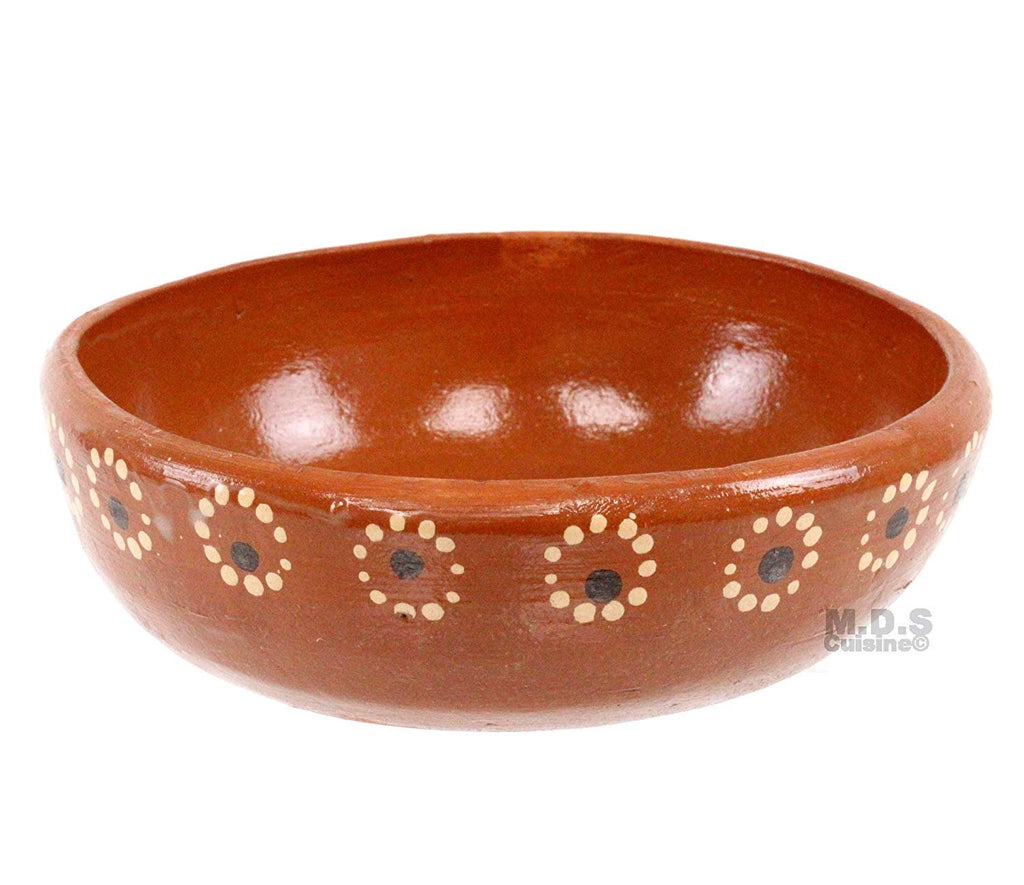This image features a close-up view of a hand-crafted wooden bowl against a plain white background, showcasing its intricate, hand-painted design. The bowl, a light brown color with hints of reddish-orange, appears to be ceramic or heavy stoneware, approximately eight inches wide and four inches tall. It has six symmetrical patterns along its sides, each consisting of a white circle made from a series of dots, enclosing a single black dot placed at varying positions within the white circle. The bowl has a reflective surface in its center, revealing four rectangular highlights likely from overhead lighting. Near the bottom right edge of the image, light gray text reads "MDS Cuisine," with a copyright mark subtly indicating the artisan’s authenticity. The bowl exhibits slight imperfections and chips, further emphasizing its handmade quality.